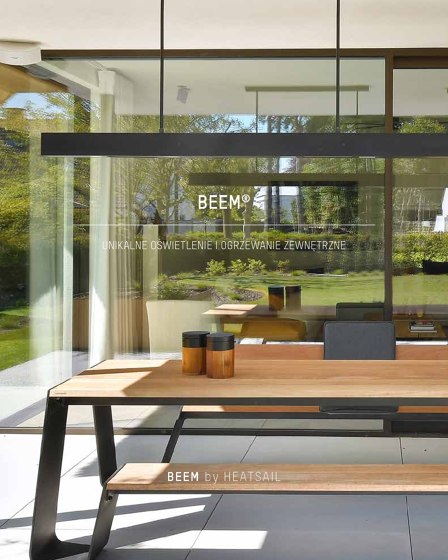This outdoor scene is set under a covered area of a building with a white ceiling. In the foreground, there's a medium-brown picnic table with black trim and legs, positioned on a stone-tiled ground. The table features two cylindrical containers with black caps, possibly coffee creamers. On the opposite side of the table, there is a seat with a black backrest. Behind the table, large glass windows offer a view into what appears to be a restaurant or store. The windows are prominently marked with "B-E-E-M" in all caps, alongside a trademark symbol. Below this, in a different language, are the words "UNIKALNE OŚWIE TLENIE I OOGRZEWANIE ZEWNĘTRZNE," which translates to unique lighting and outdoor heating. Hanging from the ceiling above the table is a rectangular black light fixture. Through the glass windows, trees and a patch of grass are visible, adding a touch of greenery to the scene. The area appears to be an atrium, offering a blend of indoor comfort in an outdoor setting.